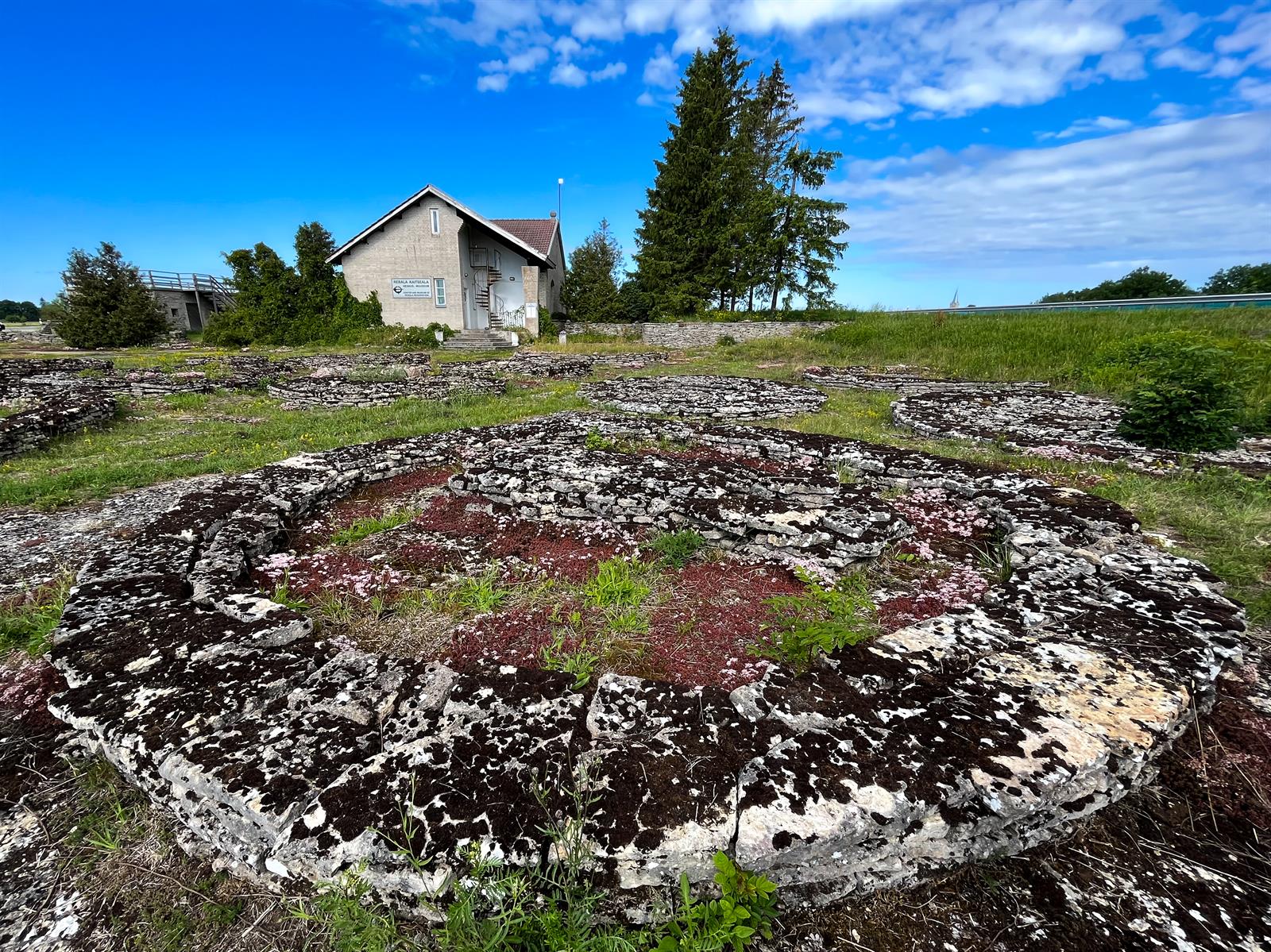The photograph captures a scenic, grassy field with a distinct building situated towards the upper left side of the image, identifiable by its triangular-shaped roof and light brown or gray walls. The building, which is likely not a house due to the presence of a visible sign on its wall, sits amidst a natural setting with scattered trees and bushes. Adding to the rustic ambiance, the foreground features numerous low, circular concrete structures, possibly old wells or similar constructs, suggesting a lack of maintenance as they are overrun with grass, dirt, and weeds. A highway railing is visible on the right-hand side, indicating the location might be alongside a road. The scene is bathed in sunlight with a blue sky dotted with fluffy, scattered clouds. The greenery extends into the distance, blending with more trees on the far right, accentuating the tranquility and remote nature of the setting.